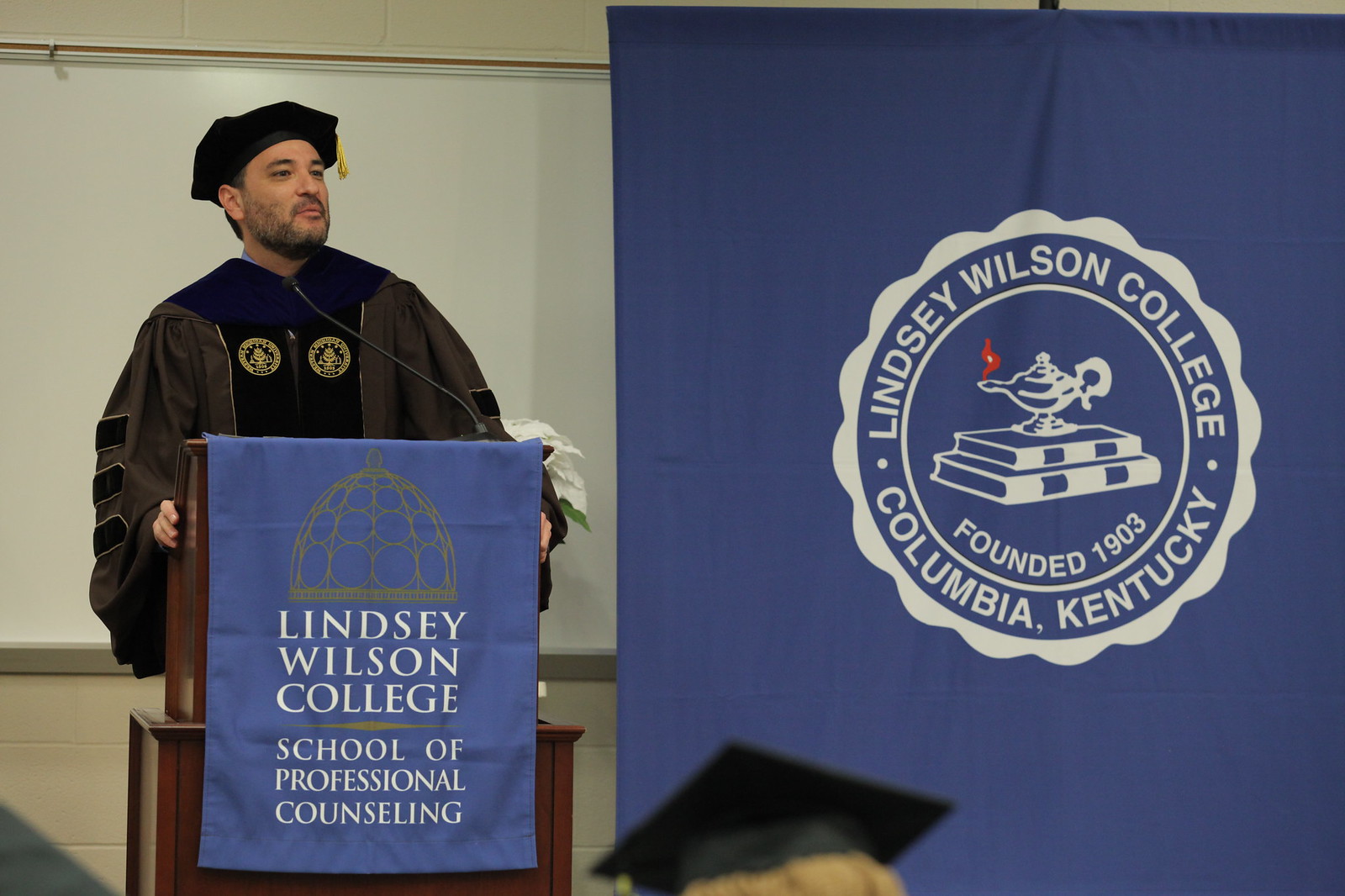This is a photograph of a white male graduate from Lindsey Wilson College School of Professional Counseling, standing at a deep wooden podium, delivering a speech. He is wearing a black and dark blue graduation gown with black velvet stripes on the sleeves and a navy blue sash. The gown features two gold emblems on either side of the velvet stripes. He is adorned with a black velvet cap and a gold tassel. The podium is draped with a navy blue banner that has white text reading "Lindsey Wilson College School of Professional Counseling." Behind him, there is a large navy blue banner with a round seal, displaying the logo of Lindsey Wilson College, Columbia, Kentucky, founded in 1903. The seal features two stacked books with an oil lamp on top, and a small red flame emerging from the lamp. The graduate appears to be in the middle of delivering an inspiring speech, gripping the podium and speaking into a microphone.